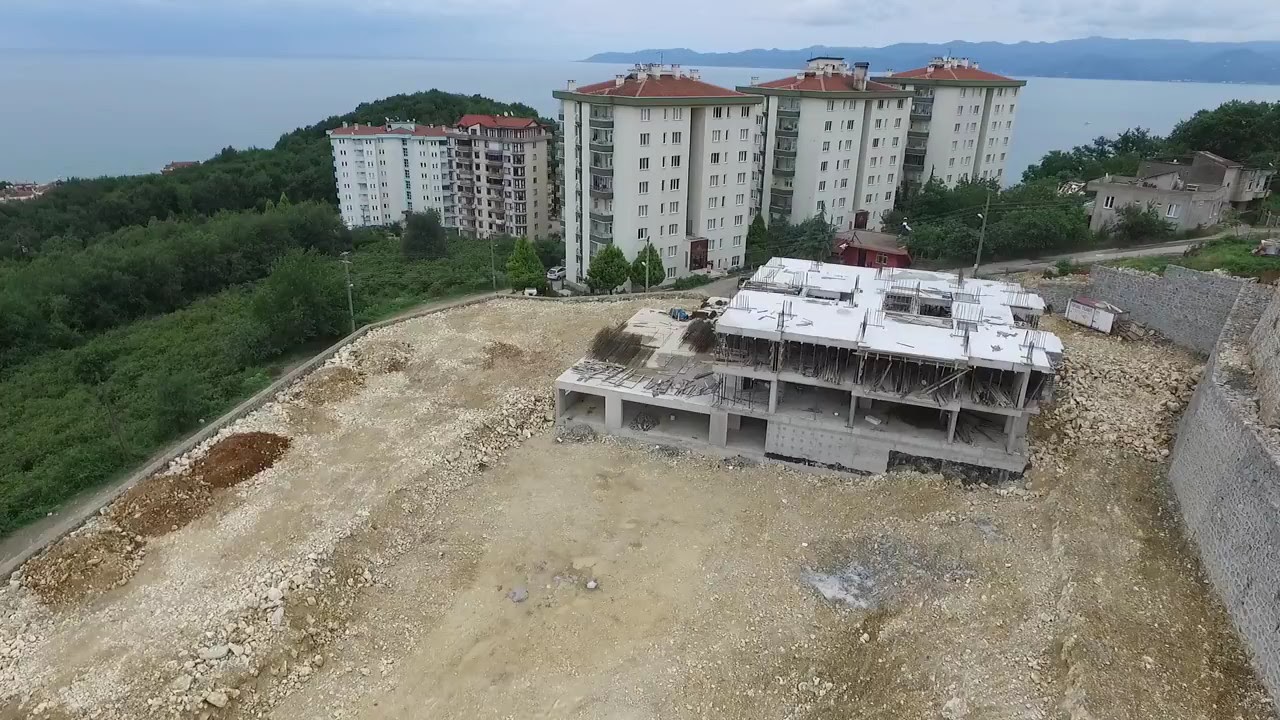The photograph, captured from an aerial drone, presents a detailed view of an active construction site on an elevated plot of land by a shoreline. The image, in landscape orientation, showcases a partly cloudy sky. At the center, a concrete building under construction is prominently displayed, revealing its three-story structure with an additional parking area to the left. The plot is rectangular and covered in beige and gray dirt, sporadically littered with mounds of gravel and rubble. Surrounding the construction site is a gray brick wall on the right, encapsulating the largely dirt-filled area. 

Beyond the construction site, a road separates the site from a cluster of high-rise buildings with white stucco exteriors and red tile roofs—likely apartments or hotels ranging from 8 to 10 stories high. These buildings are nestled on a hillside abundant with lush green vegetation. Further in the distance, a vast body of water stretches out, identifiable as a sea or ocean, with a dark blue island jutting from the horizon on the top right side of the image. The photograph embraces elements of photographic realism, capturing the serene yet industrious scene without any visible human presence.